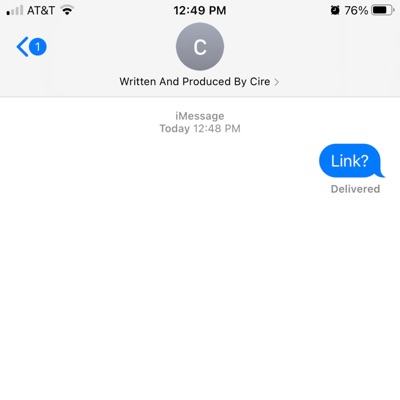The image captures the top portion of a smartphone screen encased in a wide gray banner. In the upper left corner, four signal bars are displayed, with only the first bar filled in black and the remaining three in gray. Adjacent to these bars, the carrier name "AT&T" is visible. Further along, a signal indicator shows two black bars with a gray bar on top. The time is displayed next, reading "12:49 PM," followed by an alarm clock icon and a battery indicator showing 76% charge, with the battery icon predominantly black and orientated to the right.

Below this row, there is another line containing several icons and text: a blue arrow pointing left, a blue circle with a white number "1" inside, and a large gray circle with a white letter "C" in the center. Subsequent text reads, "Written and produced by Cire" with an additional arrow pointing to the right.

In the main section of the image, which is white, the text "iMessage Today 12:48 PM" is centrally placed, immediately to the left of a blue speech bubble containing the text "Link?" with a capital "L." Below this message, the word "Delivered" appears in small, bold gray typography.